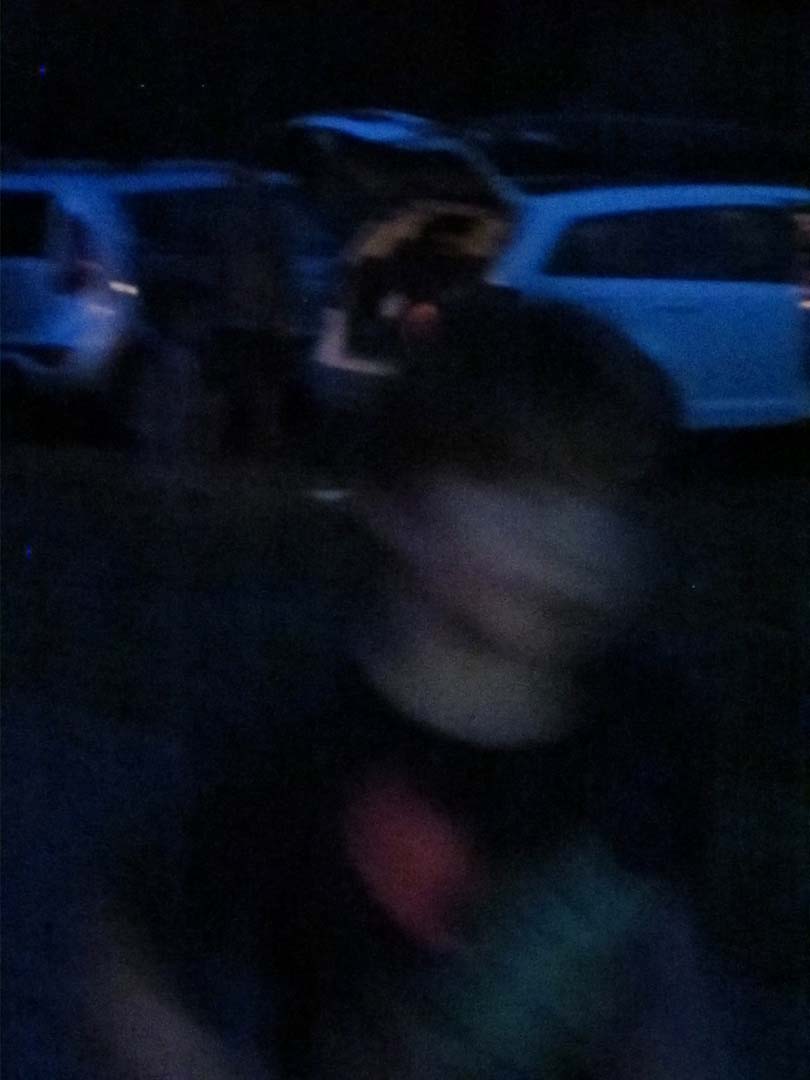The image portrays a very blurry nighttime scene, likely captured with a phone camera, featuring a young person with short dark hair standing prominently in the foreground. The person wears a black shirt adorned with a noticeable red spot on the top left and some blue text on the bottom right. In the dim and indistinct background, there are a couple of white vehicles, likely SUVs or vans, with one having its trunk open. The open trunk reveals what might be a person or additional objects, though details are obscured due to the blur. The entire image suffers from poor visibility, making finer details such as the exact actions or identities of any background figures difficult to discern. The ground varies in shading from dark to lighter gray patches, contributing to the overall hazy quality of the scene.